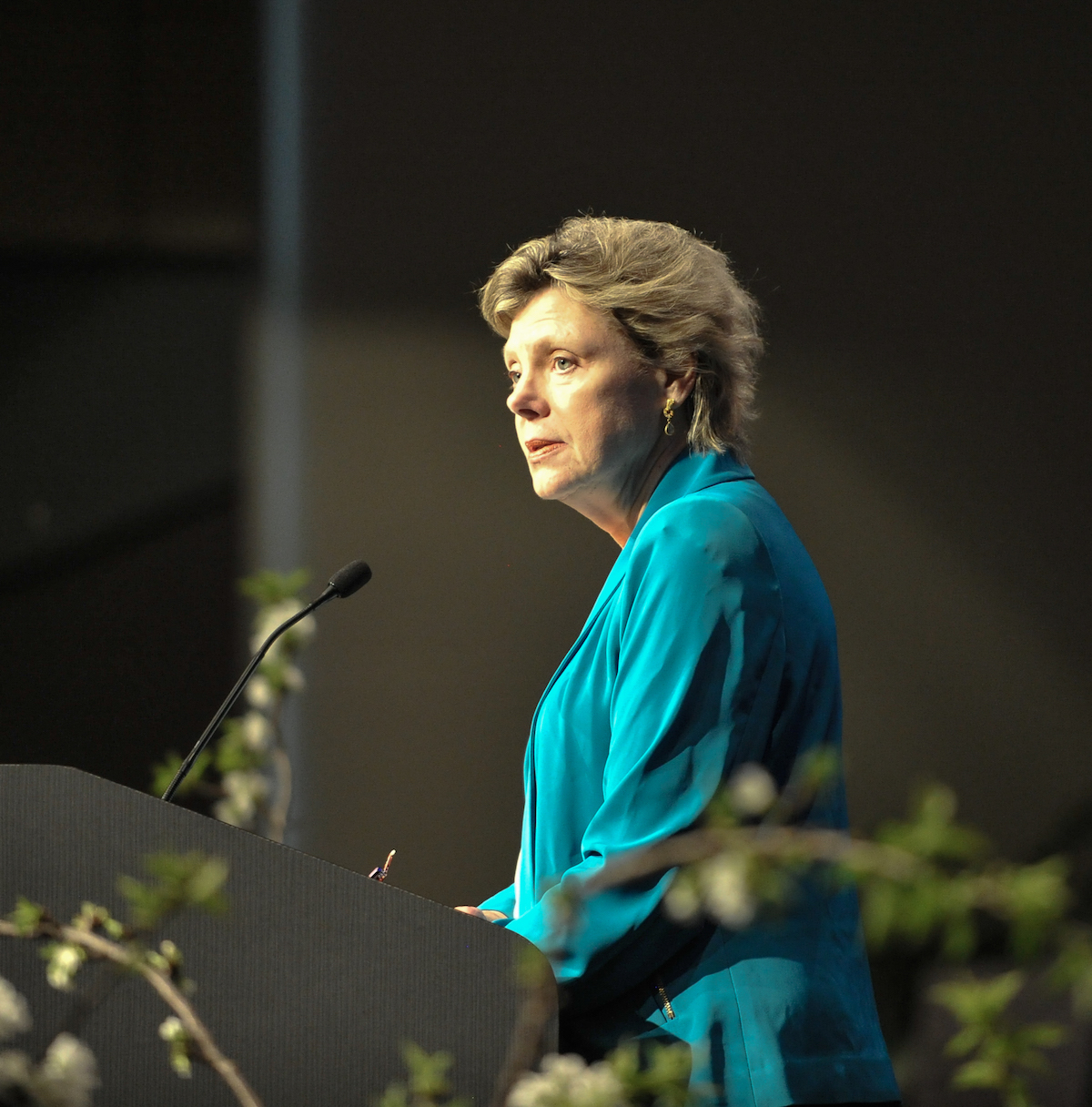In this image, we see an older woman, possibly the journalist Cokie Roberts, standing at a gray podium, speaking into a thin black microphone. She appears to be in her 60s or 70s, with short brown hair adorned with earrings, and she's wearing a formal light blue or turquoise dress or blouse. The setting seems to be indoors, possibly a lecture hall or a venue for a solemn event like a memorial or funeral, as indicated by the subdued lighting and serious expression on her face. The background is predominantly gray and slightly blurred, with the presence of small plants or trees visible both in the foreground and behind her, adding to the formal and somber atmosphere. She is positioned slightly to the left of the frame, looking out at an unseen audience, illuminated by indoor lighting.